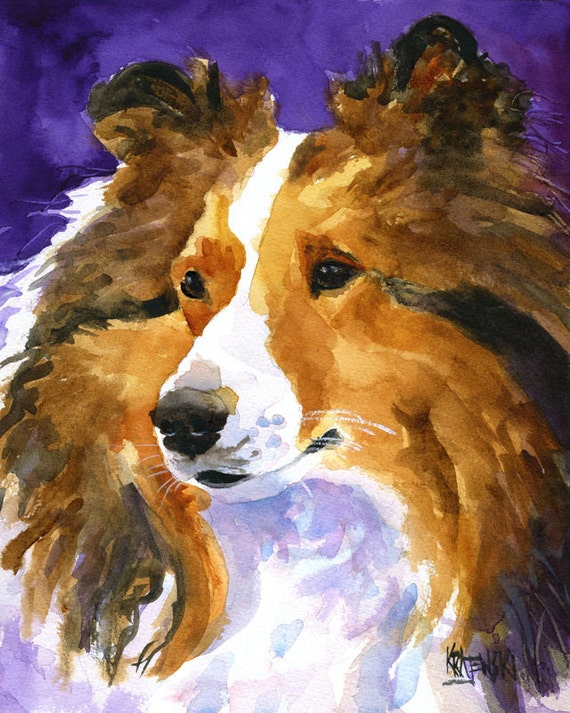A detailed watercolor painting by Anna Kronensky captures the portrait of a Border Collie. The background transitions from deep violet at the top to lighter shades of purple mingled with white towards the bottom. The focus of the artwork is the dog's face, which occupies most of the canvas. The Collie, with a slightly abstract and less realistic style, features heavy brushstrokes and muted colors. The dog's fur is primarily a rich medium brown, accentuated by shades of darker brown and black along the cheeks and ears. A distinctive white stripe runs from the forehead down to the snout and chin, contrasting with its black nose. The Collie's dark brown eyes, with black pupils, gaze off to the right, adding a sense of depth and curiosity. Each strand of fur is vividly detailed, capturing the natural texture and flow. The painting is signed at the bottom, though the signature is somewhat difficult to decipher.